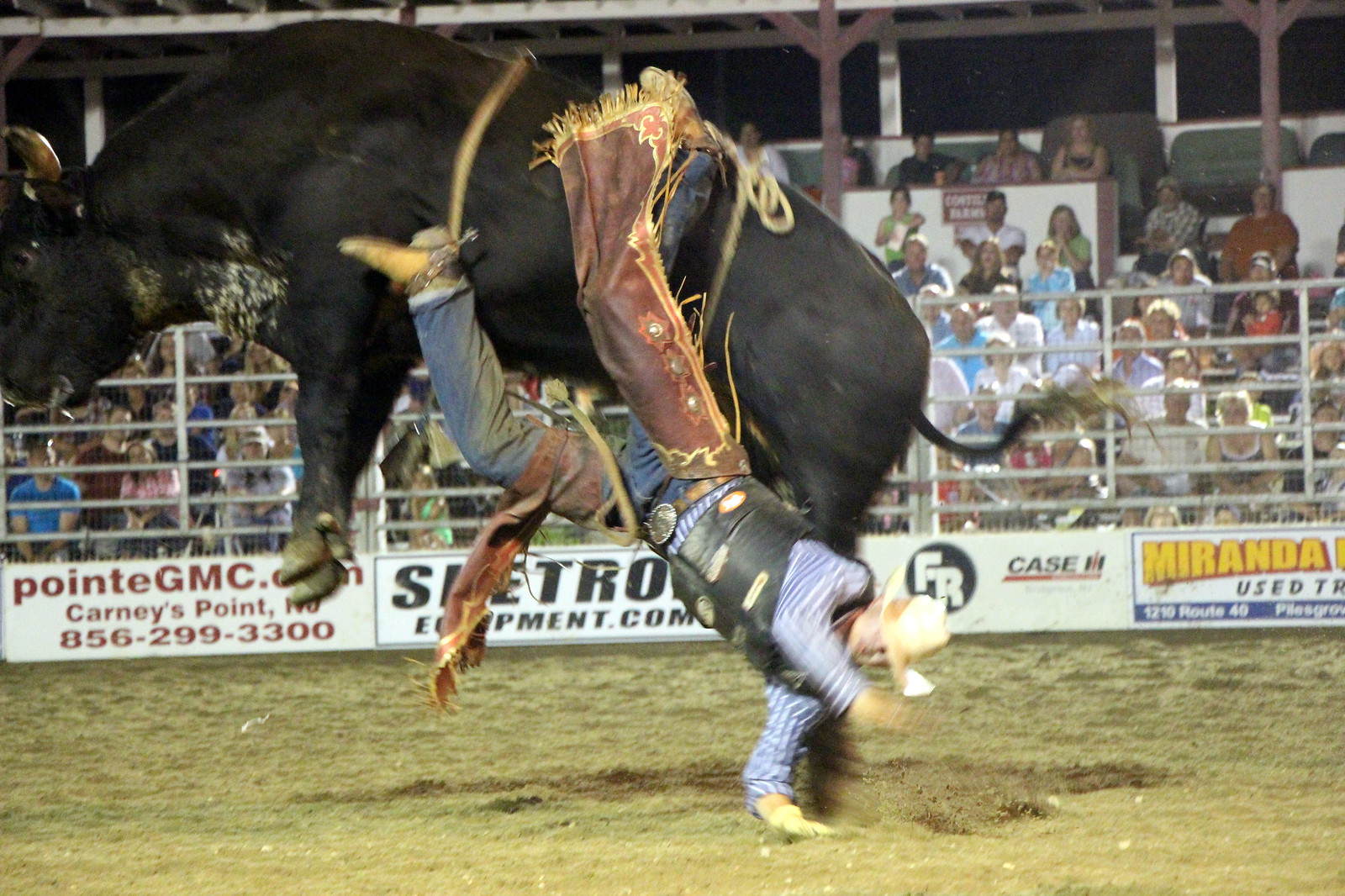The image captures a dramatic moment at a rodeo, where a cowboy, clad in brown chaps with gold fringes and a black leather vest adorned with a few patches, is being thrown off a fierce, dark black steer. The bull, with its brown horns and powerful legs kicking upward, is fully airborne, with all four hooves off the ground, facing left in the photograph. The cowboy, who is nearly upside down, appears to have his foot caught in the stirrup as he is hurled towards a surface of sawdust and sand. His cowboy hat miraculously remains on his head. A large crowd watches intently from behind a fence, with clear signage visible behind them: "Point GMC Kearney Point 856-299-3300," "Miranda Used Something," "FR Case," and "SutronEquipment.com," suggesting a typical rodeo setting.